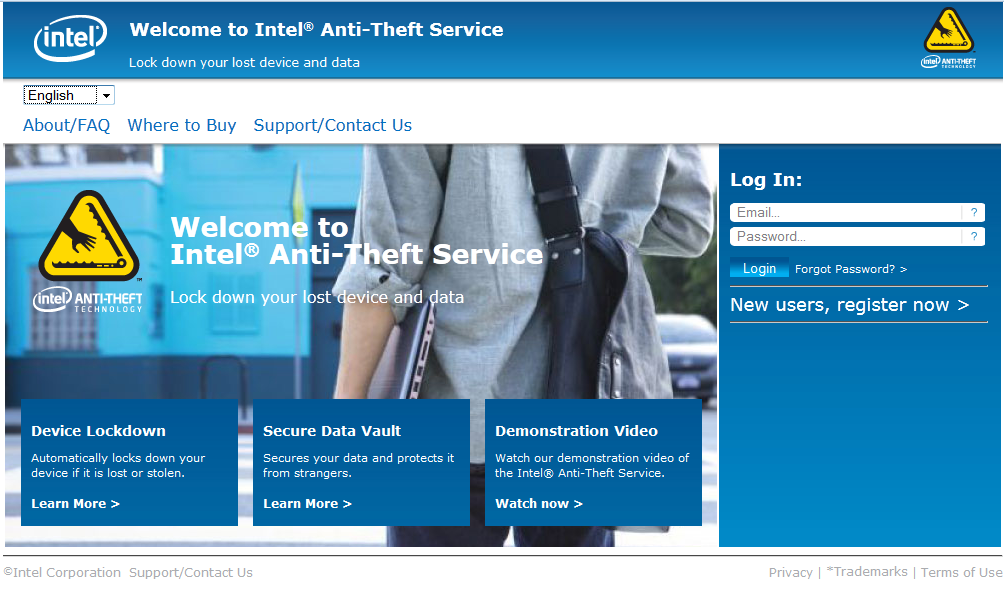Sure, here's a cleaned-up and detailed caption for the image described:

---

The launch page for Intel's Anti-Theft Service features a mixed blue and white background. At the top, a blue banner prominently displays the Intel logo, encased in a small oval, and bears the welcome message: "Welcome to Intel Anti-Theft Service. Lock down your lost device and data" in white text. To the right of this message, there is a warning icon: a triangle with rounded edges, outlined in black with a yellow interior, depicting a hand being chomped by a laptop with sharp teeth.

Directly below this section, the phrase "Intel Anti-Theft Service" appears, followed by a language selection drop-down menu displaying "English." Below the drop-down, there are four blue hyperlinks labeled: "About/FAQ," "Where to Buy," and "Support/Contact Us."

An image further down the page shows a person walking away, who could be either a man or a woman, wearing a gray shirt and black pants. The individual carries a small backpack and holds a silver laptop in their left hand. Accompanying this image, the text "Welcome to Intel Anti-Theft Service" is repeated, along with the same laptop-hand icon to the left, reinforcing the message, "Lock down your lost device and data."

Three blue boxes with white lettering are aligned below, each representing a key feature of the service: "Device Lockdown," "Secure Data Vault," and "Demonstration Video," with options to "Learn More," "Learn More," and "Watch Now," respectively.

To the right of these boxes, against a blue background, are fields and buttons for user login. The section includes input boxes for "Email" and "Password," along with buttons labeled "Login," "Forgot Password," and "New Users, Register Now."

---